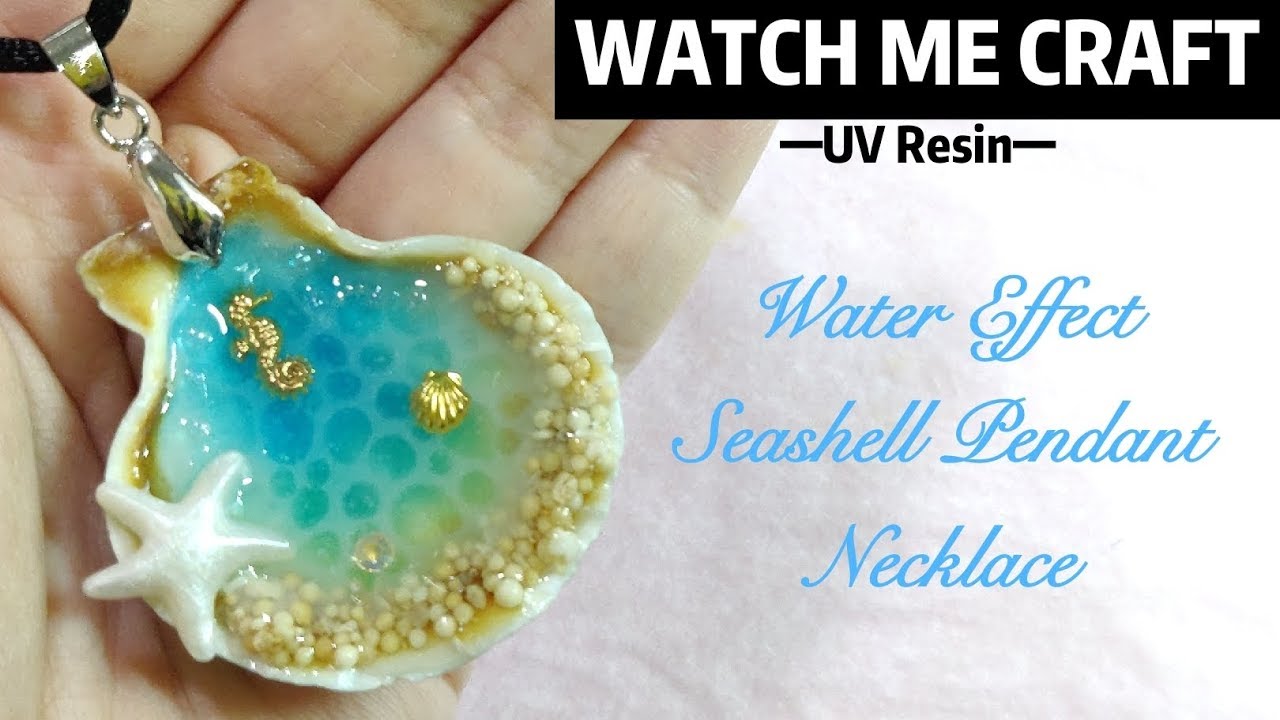In this horizontal advertisement photograph, a Caucasian hand emerges from the bottom left corner, partially displaying the fingers as they extend diagonally across the image. The hand holds a necklace featuring a black string or fabric that starts from the upper left corner, and a silver clasp connects to a silver circle. The focal point is a scallop-shaped pendant, artistically crafted to look like a miniature seascape. This pendant exhibits a water-like blue surface with gray spots at the top, adorned with a tiny white starfish on the left, a central golden seahorse, and a small gold seashell below to the right. Small bead-like stones encircle the lower edge of the scallop shell, adding texture and depth. Text in blue letters, "Water Effect," is visible to the right of the pendant. In the upper right corner, a black rectangle contains the phrase "Watch Me Craft" in white letters, accompanied by two smaller horizontal black lines with the words "UV Resin" beside them. The faint pink fabric in the background enhances the aesthetic appeal, creating an inviting, beach-like vibe. This intricate seashell pendant necklace, suggested by the text, offers a glimpse of the artistic craftsmanship involved in its making.